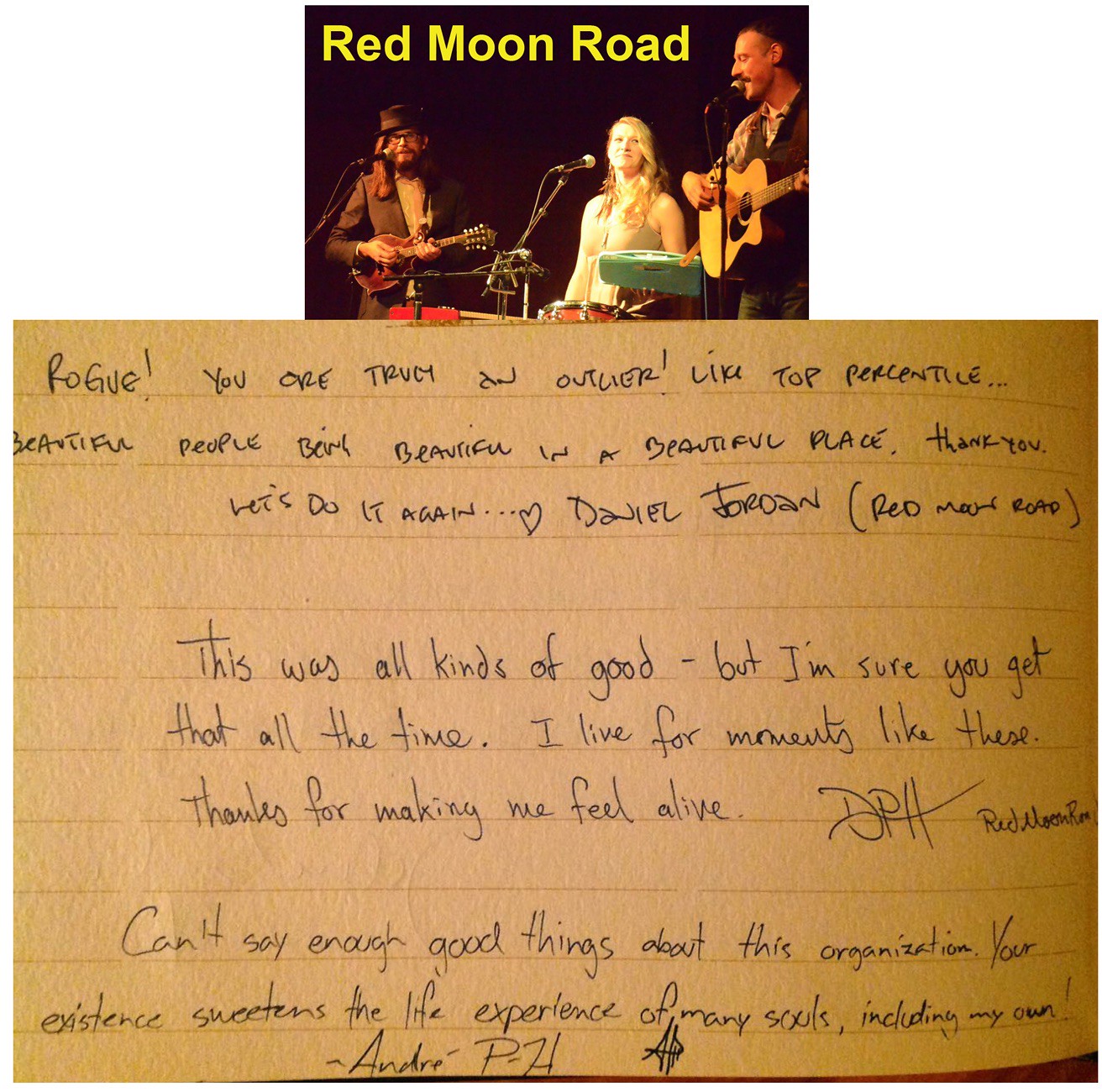The image features a three-person band called Red Moon Road, with the band’s name displayed in bright yellow writing against a dark background at the upper left-hand corner. The band comprises a man with a guitar positioned in front of a microphone, a woman sitting at a drum set, also in front of a microphone, and another man playing a smaller guitar or possibly an electric ukulele, similarly in front of a microphone. The man on the right appears taller than the others by a head. Below the image, there is a handwritten note expressing deep appreciation for the performance. The note reads: “Rogue, you are truly an outlier. Like top percentile, beautiful people being beautiful in a beautiful place. Thank you. Let's do it again. Daniel Toran, Red Moon Road.” Additional messages include: “This was all kinds of good, but I think I'm sure you get that all the time. I live for moments like these. Thanks for making me feel alive. DPH,” and “I can't say enough good things about this organization. This instance sweetens the life experience of many souls, including my own. Andre Ph.”